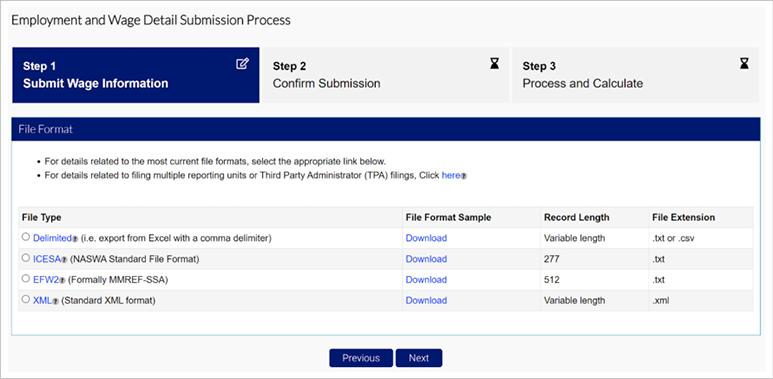The image illustrates a desktop screenshot with a white background featuring a detailed guide on the "Employment and Wage Detail Submission Process." The content is organized into three main steps and a section on acceptable file formats for submission.

The first step, "Submit Wage Information," is highlighted with an icon depicting a piece of paper and a pencil. The second step, "Confirm Submission," is shown with an hourglass icon in black text on a white background. The third step, "Process and Calculate," also features an hourglass icon and follows the same color scheme.

Below these steps, there's a section titled "File Format" displayed in a blue bar with white text. The accompanying boxes are shaded in white and gray, providing information in black and blue text depending on the context. This section explains that for detailed information related to the most current file format or filing multiple report units or third-party administrator (TPA) filings, users can click a blue hyperlink labeled "here."

The next part includes a chart listing different file types, formats, record lengths, and extensions:

1. **Delimited (Export from Excel with a comma delimiter)**
   - Action: Download
   - Record Length: Variable
   - File Extension: .txt or .csv

2. **ISA (ICESA, NASWA Standard File Format)**
   - Action: Download
   - Record Length: 277
   - File Extension: .txt

3. **EFW2 (Formerly MMREF-SSA)**
   - Action: Download
   - Record Length: 512
   - File Extension: .txt

4. **XML (Standard XML Format)**
   - Action: Download
   - Record Length: Variable
   - File Extension: .xml

This image effectively illustrates the process for uploading employment and wage data in various file formats, catering to different user requirements.